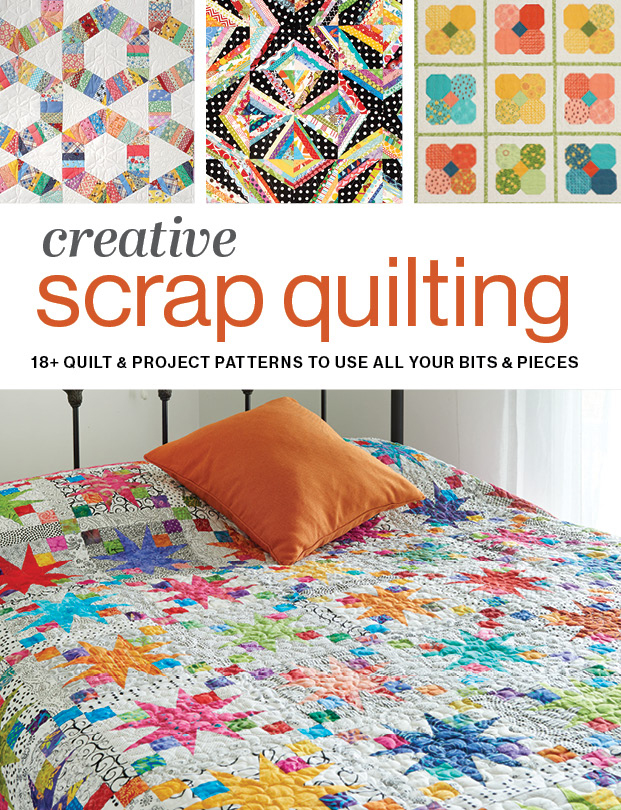The image presents the front cover of an arts and crafts magazine, focusing on creative scrap quilting. The top quarter of the cover showcases three distinct and colorful quilting patterns side by side. The first pattern features vibrant octagons or hexagons resembling a snowflake or paper towel design on a white background. The second pattern displays colorful diamonds arranged on a black and white polka dot backdrop. The third pattern highlights squares within squares, with the interior squares boasting a variety of vivid colors.

Beneath these pattern images, in the central part of the cover, bold text reads "Creative Scrap Quilting," with 'Creative' in gray and 'Scrap Quilting' in red. Further down, additional text in black announces "18+ quilt and project patterns to use all your bits and pieces."

The bottom half of the cover features a large photograph of a bed adorned with a colorful quilt made from various patterns. This quilt prominently displays blue stars, yellow, and pink elements. Positioned in the top center of the bed is an orange throw pillow. The scene is completed with a headboard consisting of simple poles extending across the top of the image, emphasizing the cozy and creative setting of the showcased quilting project.